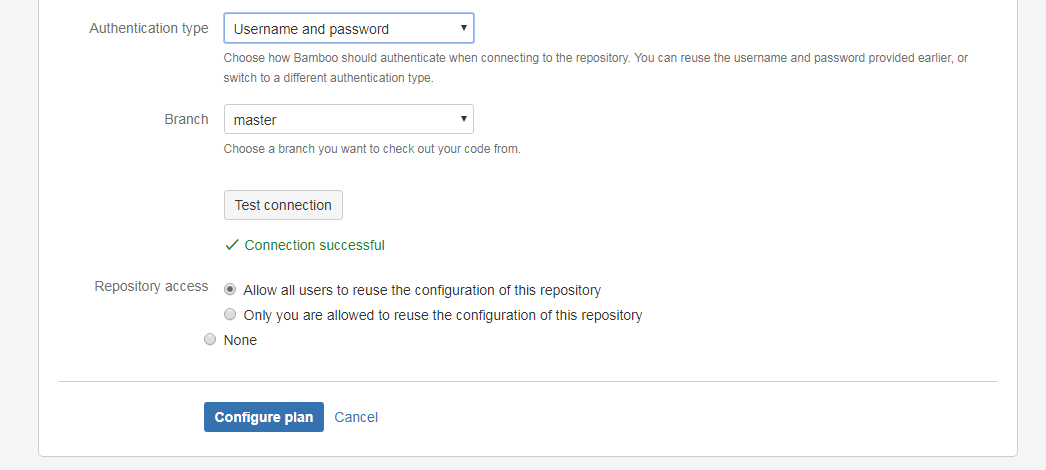This image appears to be a left-to-right horizontal screenshot, likely captured from a computer or smartphone device. The layout features a thick, medium-gray rectangle bordering the left side and a thinner strip of the same color spanning the bottom. The top edge lacks a border, revealing a subtle contrast between the white computer background and an off-white center.

At the top of the off-white section, "Authentication Type" is displayed in black text. Below it, a blue rectangular box surrounds the words "Username and Password," also in black, accompanied by a clickable downward-pointing triangle icon. Further down, relevant information about the authentication type is provided.

Next, the text "Branch Master" is followed by the instruction, "Choose a branch you want to check out on your code from." A box labeled "Test Connection" sits below, and a green checkmark indicates "Connection Successful."

The "Repository Access" section presents two options: "Allow all users to reuse the configuration of this repository" (currently selected), and "Only you are allowed to reuse the configuration of this repository." Below these options, there are two blue buttons: one for "Configure Plan" and one for "Cancel."